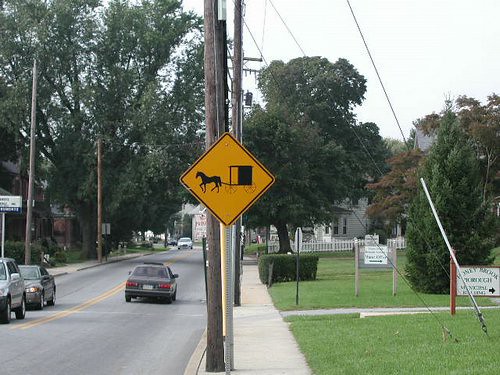This color photograph captures a detailed scene of a residential neighborhood. The image is set outdoors under a sky that is predominantly white with hints of blue. A two-way road runs through the center of the image, with a sidewalk and immaculately kept lawns on either side. Several houses line the street, with one prominently featuring a white picket fence at the far end. Numerous tall trees, especially concentrated on the left side, add a leafy, green backdrop.

There is a presence of various signage and infrastructure within the image. An orange, diamond-shaped traffic sign featuring a horse pulling a buggy draws immediate attention, positioned slightly left of center. Additional traffic signs, including a "No Parking" sign and a stop sign, are dispersed throughout. In the vicinity, signs on the lawns indicate directions to local places, with one reading "Honeybrook Borough Municipal Building." The scene also includes power poles with wiring running across, adding to the suburban feel. There are no visible people or animals in the frame, though we can see one car driving away from the viewer and two more approaching from the left edge of the image.